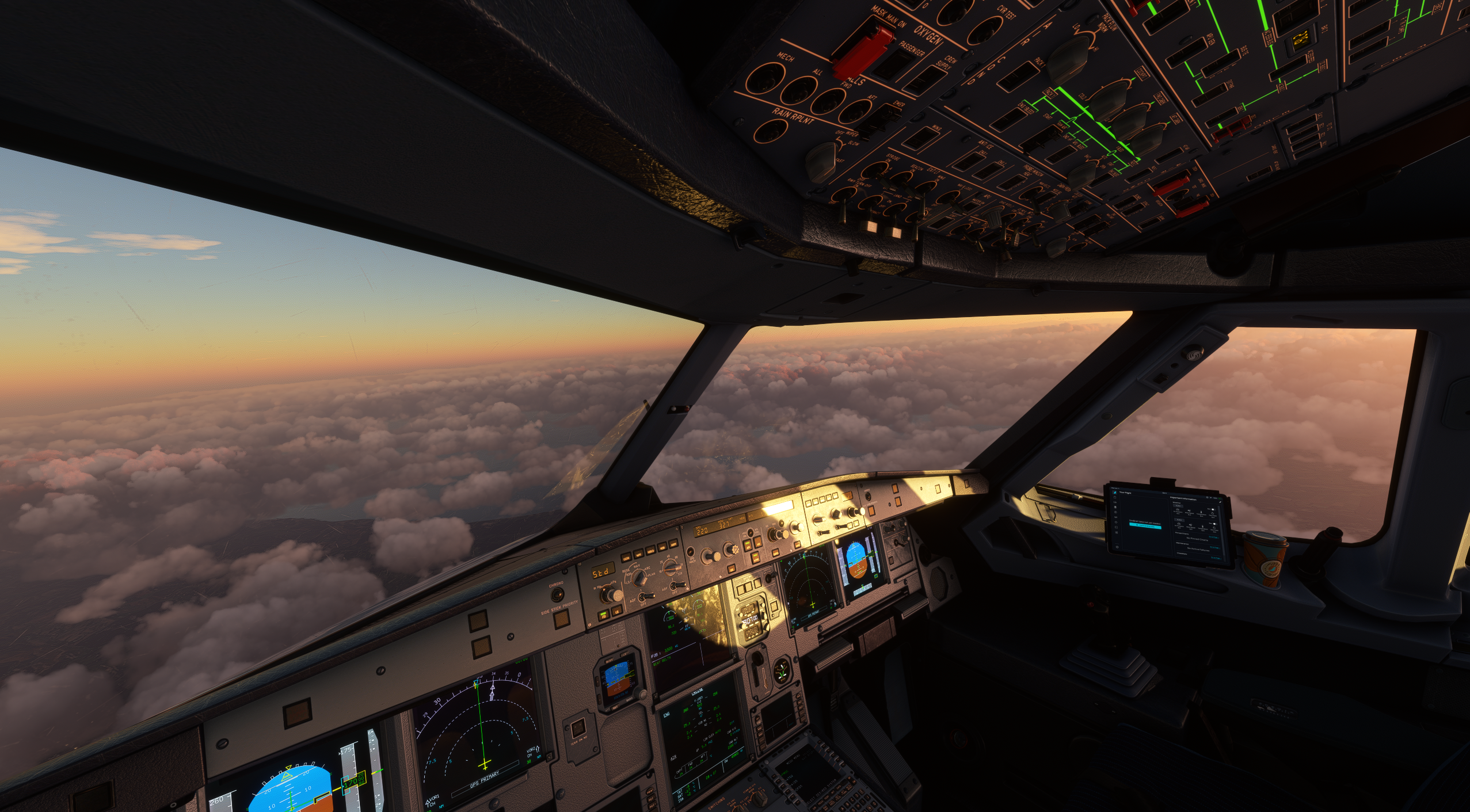This detailed, horizontal-rectangular color photograph captures the intricate interior of an airplane cockpit, as seen from the pilot or co-pilot's vantage point. The cockpit is bustling with various controls, showcasing a well-lit instrument panel adorned with an array of buttons, switches, and dials. Notably, green lights and red switches are prominently featured above, while bright blue displays add a vibrant touch to the central control panels. To the right, almost appearing like a radio, additional equipment is mounted on a shelf.

The view through the cockpit windows showcases a serene scene outside, with the aircraft soaring above a continuous blanket of white clouds. The sky above the cloud layer is a bright blue, interspersed with additional white clouds. Along the horizon, hues of bright green and orange contribute a splash of color to the scenic sky.

This detailed representation omits any text, capturing the vivid and technical essence of the cockpit’s interior against the expansive and tranquil backdrop of the sky.